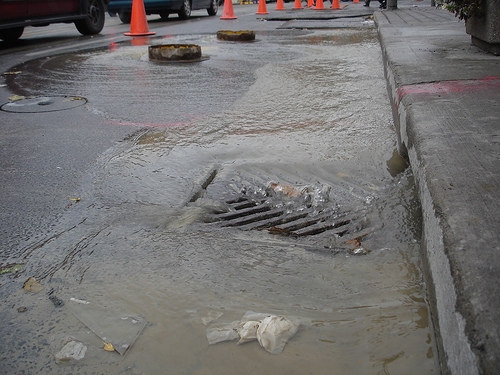The image captures a storm-flooded street with water flowing into a central sewage grate, surrounded by standing water. Trash, including what appears to be cloth or paper towel, is submerged in the flooded roadway at the foreground. To the left side of the image, a line of bright orange traffic cones partially blocks off the flooded area, extending from the top middle to the upper left of the photo. Just beyond the cones are two vehicles, visible primarily by their wheels and lower sections. Multiple raised circular entry points, metallic in appearance, also punctuate the scene, intended to facilitate further drainage if water levels rise. A sidewalk borders the street on the right, with water running off into the roadway, but no pedestrians are present.